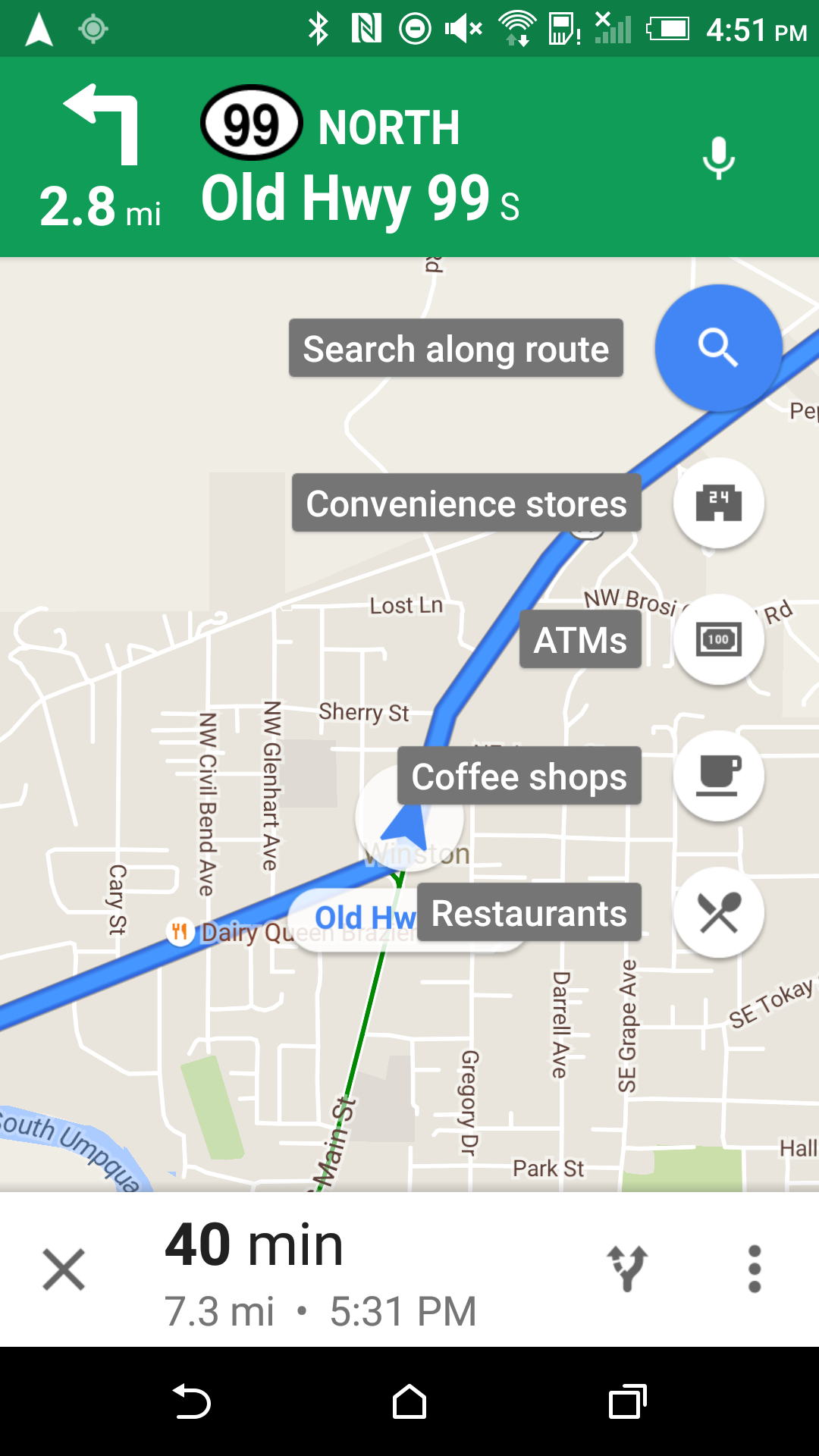The screenshot captures a detailed view of a navigation map on a mobile device. At the top of the screen, several status icons are displayed: a Bluetooth icon, a speaker symbol with the volume turned off, a Wi-Fi icon showing no signal bars, and a battery indicator with approximately 75% charge. The time displayed is 4:51 PM. There is also a back arrow pointing to the left and a distance indicator showing 2.8 miles.

In the main map section, the primary route is highlighted in blue, leading the way on North Old Highway 99. In the top-right corner of the map, there is a white circle with a black outline containing the number "99." The map, which has a gray color scheme, indicates that the route will take 40 minutes to cover 7.3 miles, with an expected arrival time of 5:31 PM.

A blue circle featuring a magnifying glass icon is displayed along the route with the option "Search along route" and several categories listed: convenience stores, ATMs, coffee shops, and restaurants. Each category is accompanied by its respective icon: a coffee cup and saucer for coffee shops and a fork and knife for restaurants.